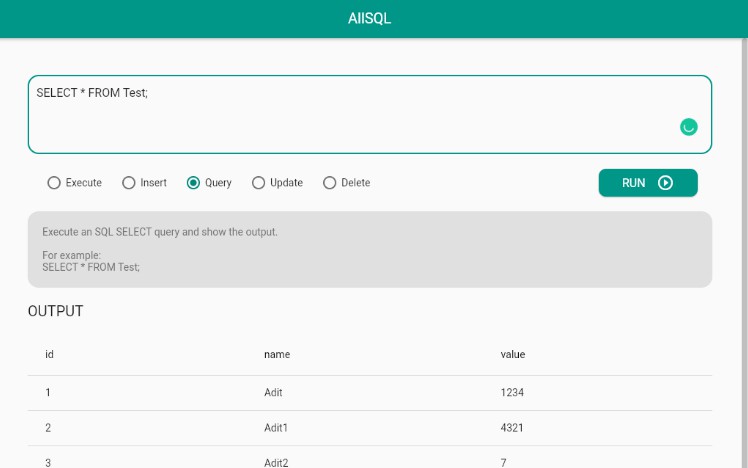The image features a predominantly white background accented by a teal banner at the top and a gradient green base. In the center of the teal banner, bold white capital letters spell out "AIISQL." Immediately below this, a green banner, matching the color of the teal, displays an outlined message in capital letters: "SELECT * FROM Test;." The section highlights "SELECT" and "FROM" in full uppercase, while "Test" features only the first letter capitalized, followed by a semicolon.

On the right side of the image, a small green circle, consistent in color with the teal, encases a simple smiley face, with the smile itself offset to one side. 

The primary white background contains a list of database commands, each preceded by a small circle: EXECUTE, INSERT, QUERY, UPDATE, DELETE—all with initial capital letters. Notably, a dot is placed within the circle next to the word "QUERY," indicating selection.

Finally, a gray banner at the bottom offers a succinct tutorial: "EXECUTE an SQL SELECT query and show the output. For example, SELECT * FROM test."